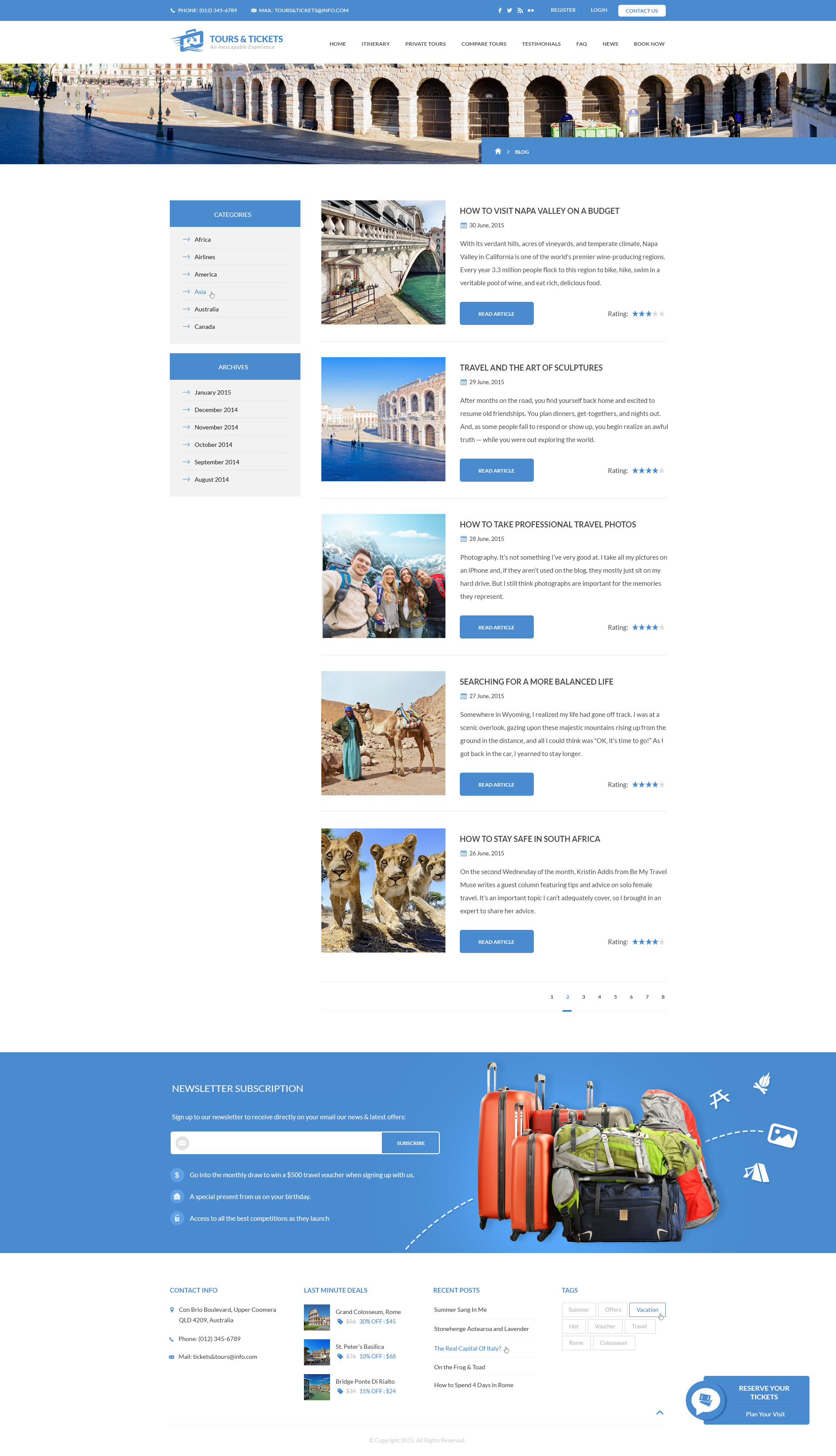Here is a detailed, cleaned-up caption for the image:

---

The image shows the lower section of a web page, likely captured from a mobile phone, featuring content related to travel, given the "Tours and Tickets" site name. At the bottom of the page, there is a subscription banner for a newsletter. Surrounding this banner are images including suitcases, bags, and small thumbnail photos that appear to be users of the website. These thumbnails are barely discernible but suggest past interactions with the site. In the middle section of the page, there are several small photographs: one depicts a person standing beside a camel in a desert setting, another shows what appears to be a group of children—two boys and two girls—playing in the snow. Additionally, there is an image of a serene canal scene, featuring a narrow waterway with a bridge overhead and a tunnel for boats to pass through. The overall page layout is cluttered, making the text and smaller details hard to read.

---

This revised caption provides a comprehensive yet clear overview of the various elements visible in the image, enhancing understanding for the reader.